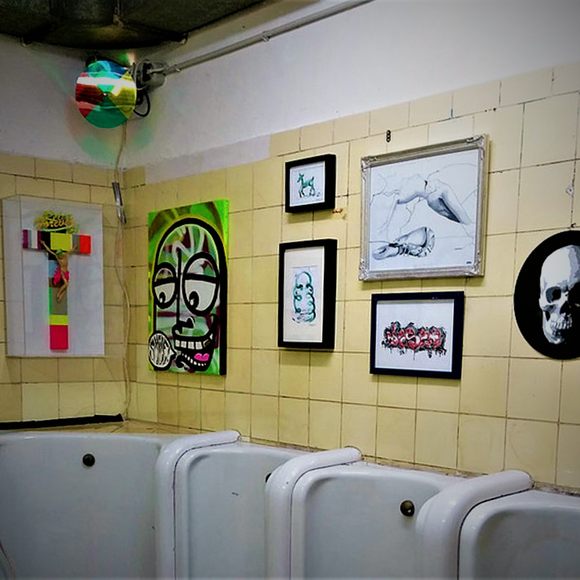The image captures the interior of a room that appears to be a male restroom, featuring multiple urinals of varying sizes lined up against a wall. The urinals are white and include one notably large, one small, and another slightly larger one, all detailed with small knobs at their center. The back wall is tiled with dingy, gross-looking yellow tiles covering approximately two-thirds of the way up, transitioning to a plain white wall at the top.

In the left corner of this tiled area hangs a vibrant, multicolored cross with a crucified Jesus figure. This cross is adorned with various colors such as gold, red, and green and includes some indistinguishable yellow lettering at the top. Above the cross, a circular symbol segmented into quarters of yellow, blue, green, and red is partially visible.

To the right of the cross hangs a green art piece, possibly spray painted, featuring a cartoonish, bald head with a slightly open mouth, possibly with an illegible speech bubble. Next to this piece is a series of framed artworks, including:
1. A balloon animal in a small rectangular frame.
2. A vertical rectangular frame depicting what seems to be a cloud.
3. A large square frame containing what looks like black and white fingers.
4. Beneath this, a rectangular photo with weird squiggly lines in red.
5. Finally, on the far right, a circular picture with a black backdrop featuring a white skull.

Each of these artworks is set against the yellow tiled wall, creating a stark contrast with their colorful and detailed depictions.